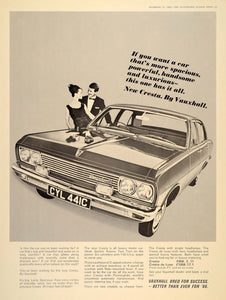This is a vintage black and white advertisement, likely from the 1950s, featuring a car dealership's promotion for a Vauxhall New Cresta. The image captures a front view of an older, four-door sedan with a British license plate reading CYL 441C. The car is notable for its four headlights and two spotlights, and "Vauxhall" is visible on the grille. To the right of the car, a well-dressed couple prepares to enter; the man is in a tuxedo with his arm around the woman, who wears a formal nightdress and has her hair in a bun. The ad includes black text in the upper right corner proclaiming, "If you want a car that’s more spacious, powerful, handsome, and luxurious, this has it all. New Cresta by Vauxhall." Additional text appears below, resembling an article, but its fine print is unreadable.